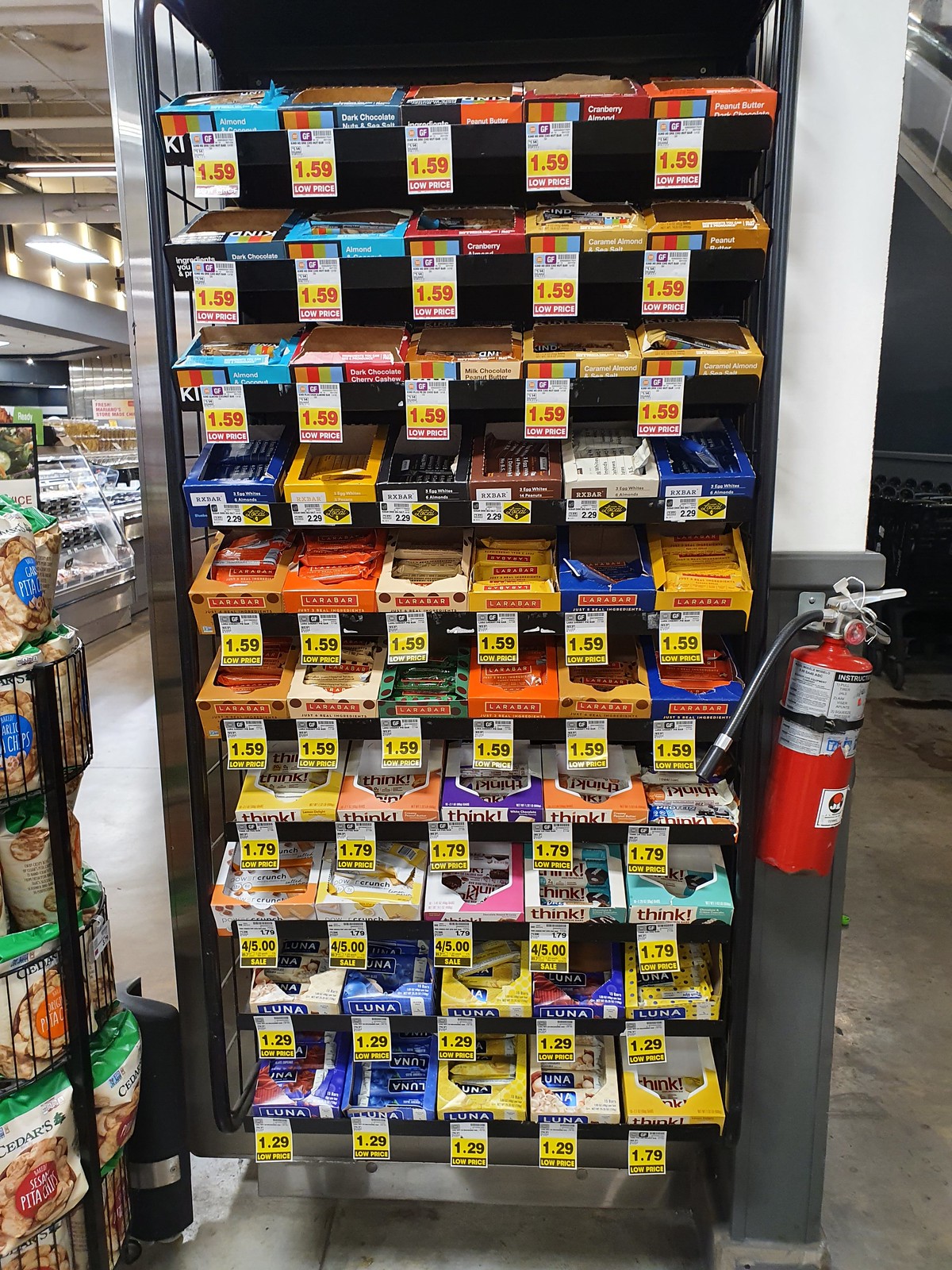In this vertically-oriented rectangular image, we are looking at a neatly organized end cap of a market aisle. The end cap is dedicated entirely to nutritional bars and consists of approximately eight or nine rows of various brands and flavors.

At the very top, we see an assortment of Kind bars, prominently featuring flavors such as Dark Chocolate Nuts & Sea Salt, Peanut Butter, and Cranberry. Just below, another row of Kind bars showcases Caramel Almond & Sea Salt and Dark Chocolate Almond varieties.

The third row continues with Kind bars, displaying flavors like Caramel Almond on the right, Almond & Coconut on the left, and Dark Chocolate Cherry Cashew situated in the center. 

The brand transitions in the fourth row to RX bars, featuring a diverse selection of colorful boxes in blue, yellow, black, brown, and white. The front of these boxes highlights key ingredients like egg whites and almonds.

In the row beneath, we find Larabars boxed in a spectrum of colors including brown, orange, beige, yellow, and dark blue, representing a variety of flavors. Following this, a subsequent row of Larabars is primarily light blue and green.

The final two rows showcase Think brand nutritional bars, followed by the last two rows filled with Luna bars. The black wire casing of the end cap allows for an open view of the remainder of the store in the background, contributing to a sense of space and accessibility.